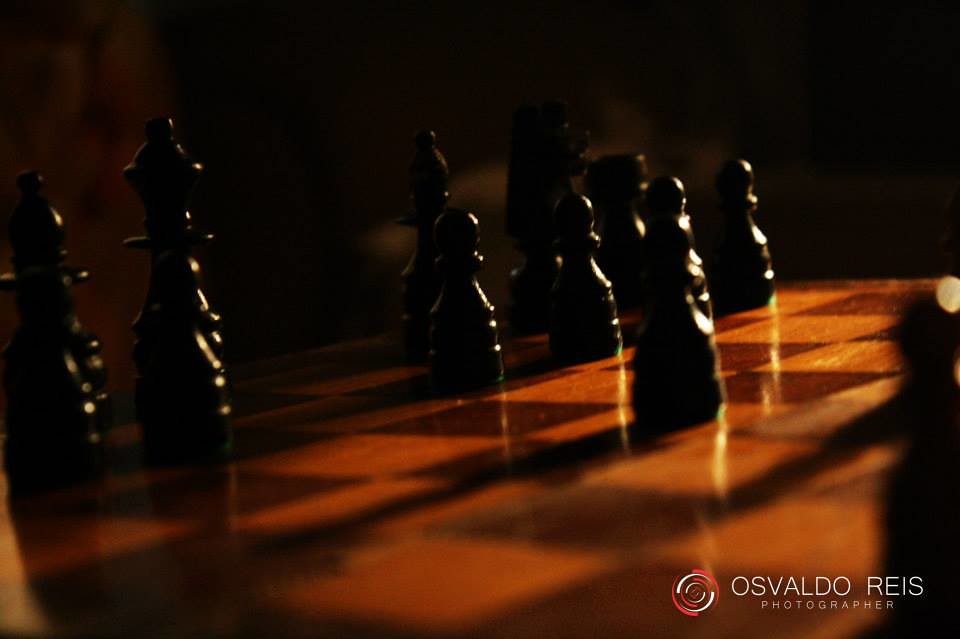This close-up image captures the black pieces on a partially visible chessboard, which features alternating dark brown and light brown squares. Highlighted by sunlight streaming in from a window, the scene is set against a dark, shadowy background. On the farthest back line of the board, starting from the left, a bishop stands on a dark brown square, followed by a king or queen on another dark square. In front of the bishop, a pawn occupies a dark brown square, with another pawn to its left where the knight would be positioned in an original setup. Moving right, there is a notable space between the king or queen and another bishop, followed by a knight and a rook in the corner. Four pawns are aligned in front of the rook, knight, bishop, and the empty square respectively. Towards the right, three squares ahead of the king or queen, a pawn rests on a light brown square. In the bottom right corner of the image, a faint, blurry object—potentially a white piece—can be seen, alongside an insignia and the white text "Osvaldo Ruiz, photographer."